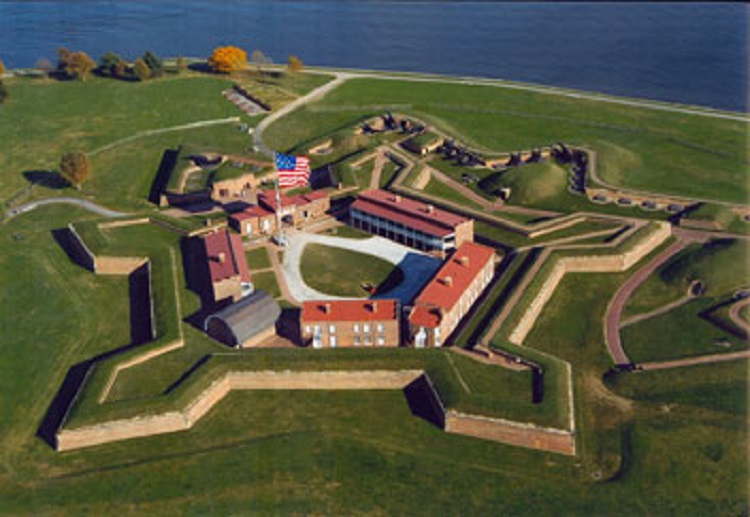This detailed aerial view captures a manicured green landscape featuring a distinctive pentagon-shaped arrangement of reddish-orange roofed buildings. These buildings, arranged in a symmetrical pentagonal layout, are surrounded by a well-maintained lawn with low-cut grass and bordered by hedges atop a brown wall. In the center of this configuration, a tall flagpole proudly displays an American flag. The scene also features a raised star-shaped guard wall enclosing the pentagon, adding to the geometric precision of the area. The upper part of the image showcases a bright blue water body, possibly an ocean, with trees lining the shore, enhancing the serene and organized aesthetic of this daytime landscape. The surrounding sunlight highlights the meticulous attention to detail in the upkeep of the grounds, suggesting a space of importance, such as a military installation or government complex.